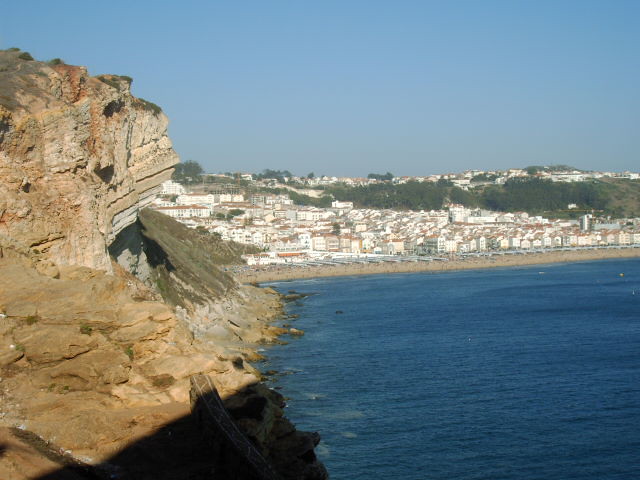The image captures a picturesque seaside village with a stunning view of a rocky cliff on the left side, contrasting against the deep blue ocean that stretches across the bottom right portion of the photo. Waves gently lap against the shore, which extends into a long stretch of sandy beach. Along this beach are various chairs, and beyond them, a charming village comprised of numerous small, white houses and storefronts. The village spreads across the lower hillside peppered with verdant trees. The upper portion of the image showcases a clear, expansive blue sky, framing the entire peaceful coastal scene. The colors are vibrant, with hues of blue from the ocean and sky, tans and browns from the cliffs, and greens from the trees, adding to the idyllic outdoor midday setting.